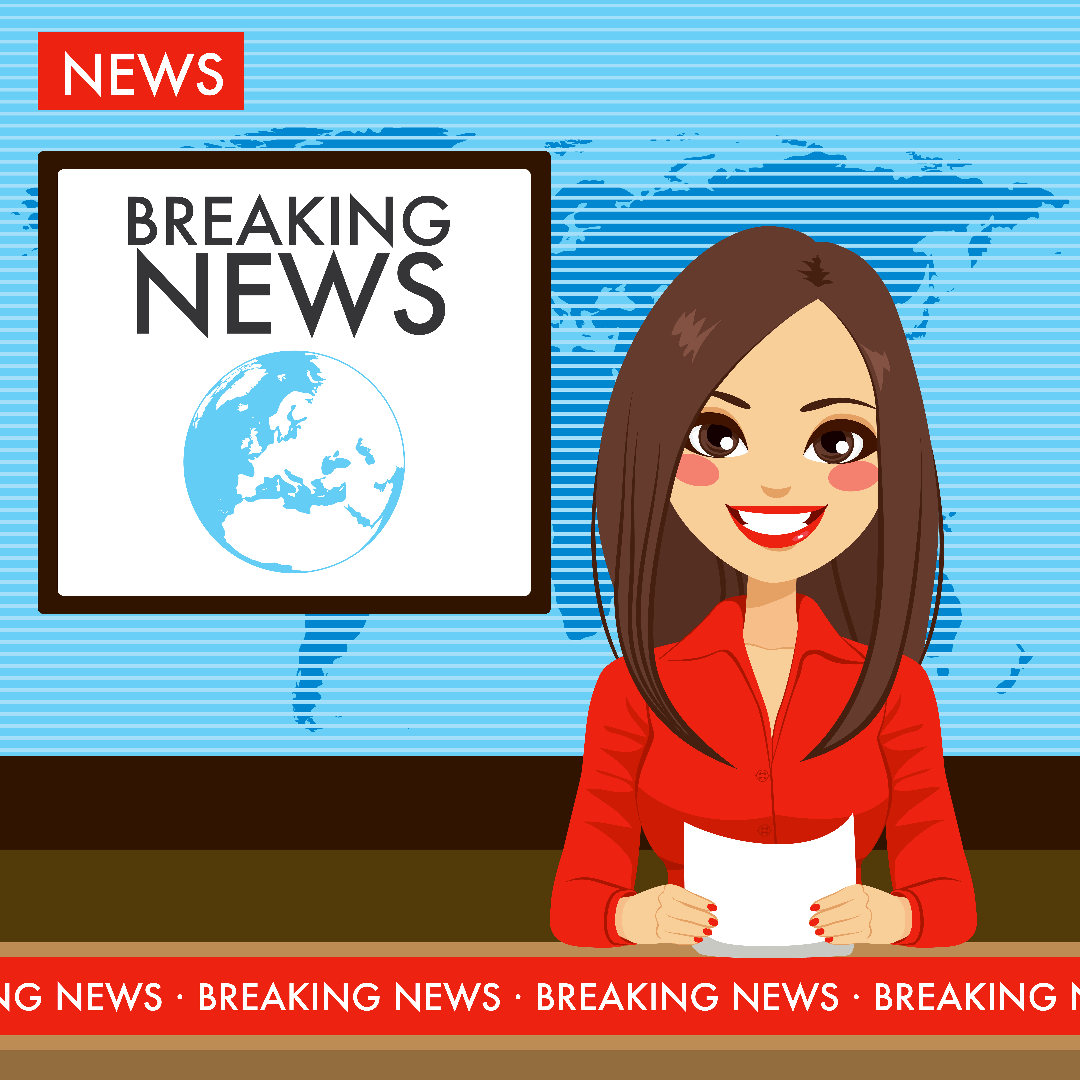This detailed cartoon illustration depicts a cheerful news anchor at a news desk, delivering breaking news. The news anchor, a woman with long, straight brown hair that falls below her shoulders, is adorned with rosy cheeks, brown eyes, and bright red lips. She is wearing a red blazer with a collared top and has matching red nail polish on her fingers, which grasp a white sheet of paper. 

In the upper left corner of the image, there’s a small red banner with the word 'NEWS' in bold white letters. Directly below this, a larger white square framed in black displays the words 'BREAKING NEWS' accompanied by an image of a globe, symbolizing global coverage. The top background features a world map in darker blue, accentuated by white lines, all set against a blue backdrop.

Adding to the urgency of the scene, a bright red banner stretches across the bottom of the screen, repeatedly flashing the phrase "BREAKING NEWS" in white capital letters. The anchor sits at a brown desk, blending into the overall professional yet vibrant atmosphere of the illustration. The entire backdrop and elements, including the maps and globes, underscore the global importance and timeliness of the news being delivered.